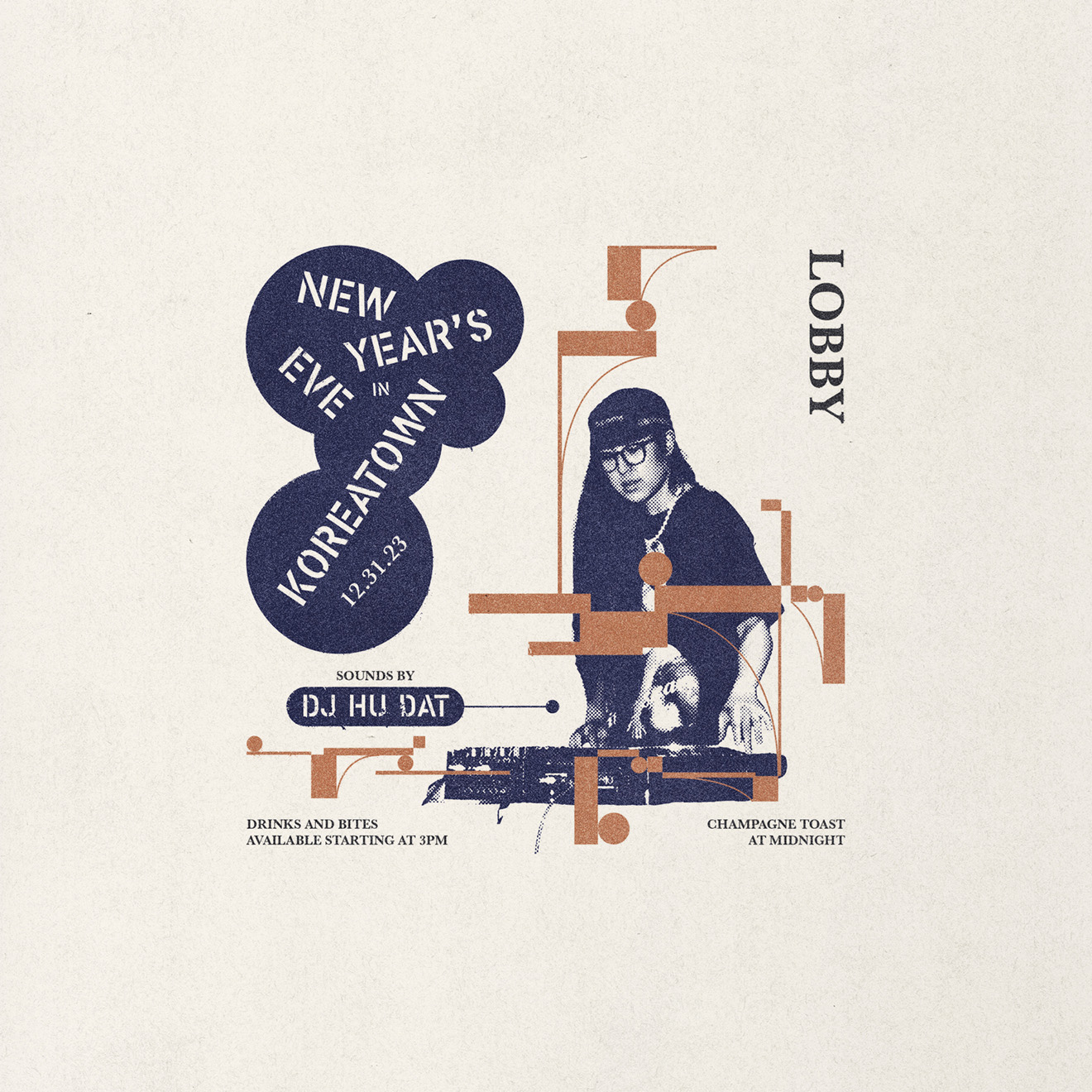This image is a square poster with an eggshell, off-white background. On the left side, a series of blue bubbles form a backdrop for stenciled navy text that reads, "New Year's Eve in Koreatown, 12-31-23." Below this, in white capital letters, it says, "Sounds by DJHUDAT," spelling out H-U-D-A-T. DJHUDAT herself appears on the right side, with long dark hair, glasses, and a pearl necklace, standing behind DJ equipment with both hands on the controls. She is wearing a black t-shirt with a print on it. The poster includes further text: "Lobby" at the top right, and at the bottom, "Drinks and Bites available starting at 3 p.m., Champagne Toast at midnight." Various simple brown geometrical patterns—rectangles, lines, and circles—are overlaid across the image, adding an abstract decorative element.